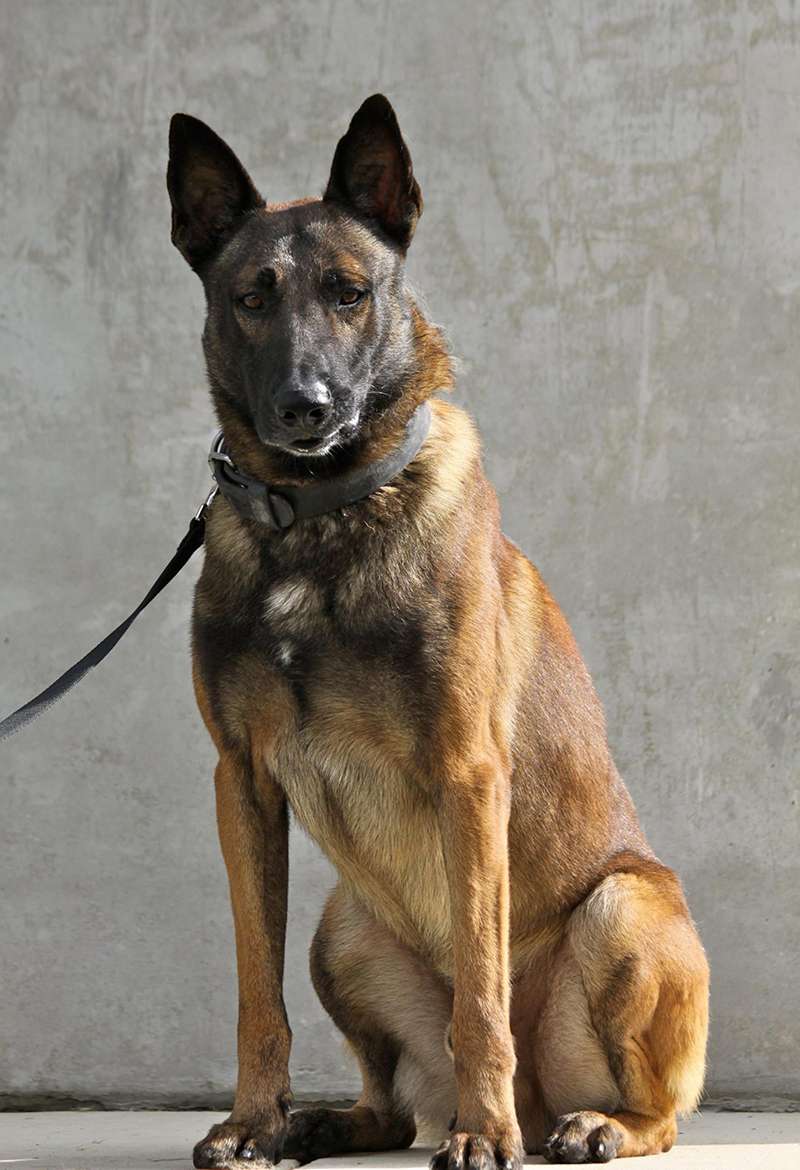This photographic image captures a poised German Shepherd seated upright on a concrete floor against a grey concrete wall. The dog, characterized by its muscular build and extended front legs, exudes both strength and attentiveness. Its fur transitions from dark grey and brown on its head to a golden brown along its body, lightening to a tan shade towards its legs. The German Shepherd's ears are pointed sharply upwards, and its expressive brown eyes look directly into the camera, capturing a hint of concern with its close-set eyebrows. A black leash hangs from a thick grey collar around its neck, trailing off to the left side of the photograph. Reflective metal bindings on the collar and leash catch the sunlight, which highlights the dog's shiny nose and enhances the textures of its fur. The minimalist and grungy backdrop of the grey wall, interspersed with faint brown lines and swirls, emphasizes the dog's prominent and striking appearance.